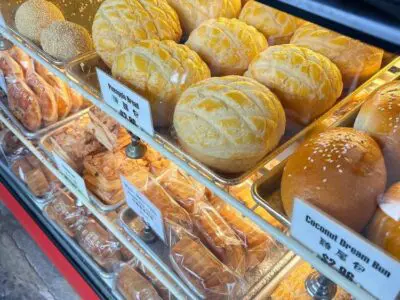This image captures a detailed, top-down perspective of a bakery display case filled with various pastries and bread items. The photo focuses on three rows of baked goods. The top row prominently features unwrapped, fresh rolls and buns, including one labeled "Coconut Dream Bun" priced at $2.88 with accompanying text in an Asian script. The middle and bottom rows contain more pastries, some resembling danishes and cinnamon rolls, with several items wrapped in plastic packaging. The pastries exhibit shades of brown and tan, indicative of their baked nature, with no bright or colorful elements present. The display case includes a distinctive red stripe along the bottom left, and a black section with a white shadowy line at the top right. The overall composition suggests a well-lit, organized array of freshly baked items ready for purchase.